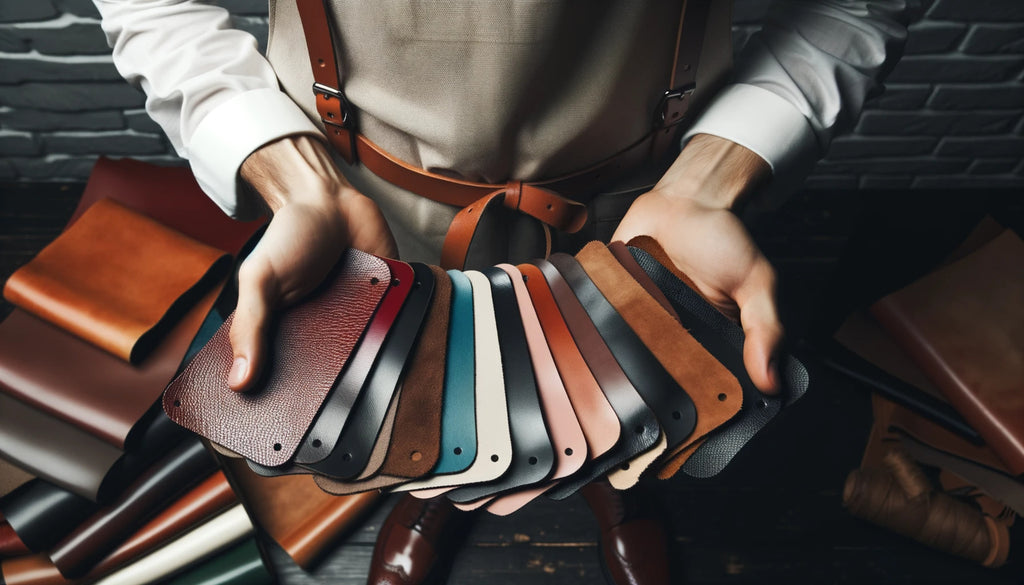In the image, we see an AI-generated man, depicted from just below his chest to his feet, standing against a gray brick-mortared background. He is wearing a white shirt, visible only at the sleeves, underneath a brown apron-like garment that has matching brown suspenders and a belt. The man is holding up an array of colorful leather samples—red, black, brown, green, white, pink, peach, orange, and more—in his white hands. These leather samples, approximately the size of credit cards and featuring holes in their corners, are fanned out in front of him. Additionally, large folded pieces of leather in various colors are visible around him. The man's outfit is completed with brown leather dress shoes, hinting at a setting inside a leather workshop or shop.